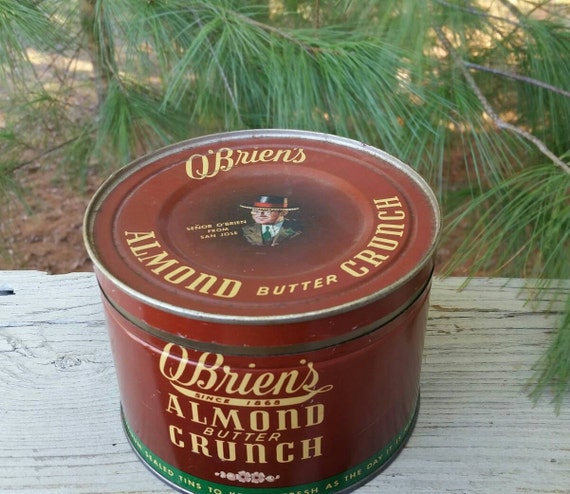This photograph captures an old-fashioned, dark red tin can of O'Brien's Almond Butter Crunch, prominently displayed on a wooden bench. The image is taken from a slightly elevated side angle, allowing a clear view of both the top and the front of the tin. The top lid features yellow lettering reading "O'Brien's Almond Butter Crunch" encircling an illustration of a man in a gray suit and black hat accented with red. The front of the tin showcases the text "O'Brien's, Since 1860, Almond Butter Crunch" in red and yellow lettering, bordered at the bottom by a thin green line. The backdrop reveals a natural setting with scattered pine needles and some parts of a pine tree visible, enhancing the rustic and timeless feel of the scene.